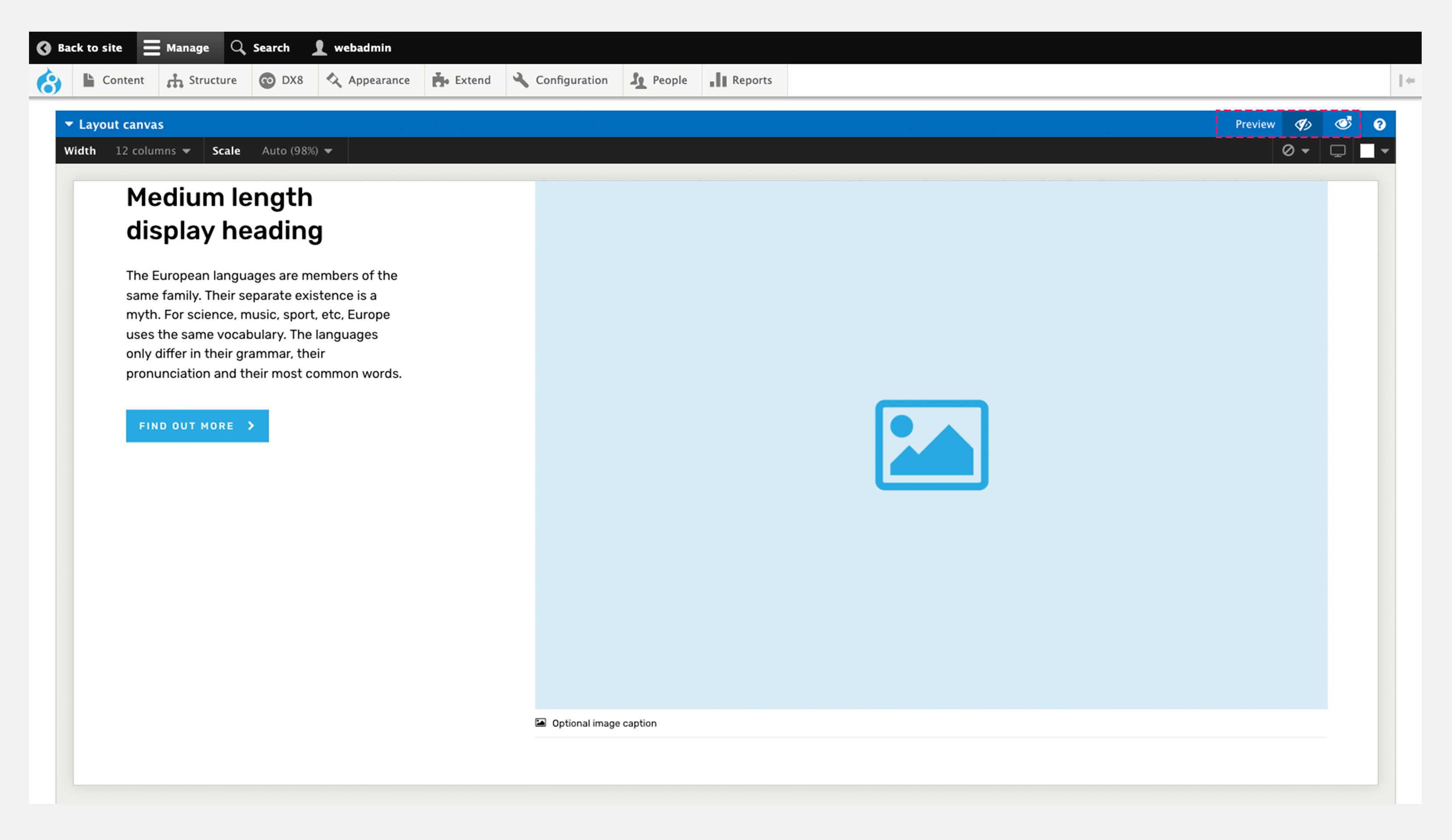In this image, the background is gray with an upper banner in black, featuring very small white lettering. The subsequent section consists of a bluish image displaying the number 8, and gray font that reads "Content Structure DX8." Below this, various categories are listed: Appearance, Extend, Configuration, People, Reports. On the left side is a layout canvas, while the right side has the word "Preview" in small letters. 

The next section features a black background with faded white font. Below this, there is a white background with medium-length black font on the left that reads: "The European language." In tiny letters below, it states: "Languages are members of the same family. A separate existence is a myth. For science, music, sport, etc. Europe uses the same vocabulary. The languages only differ in their grammar, their pronunciation, and their most common words." 

Further below, a blue text with an arrow pointing to the right invites the viewer to "Find out more." On the right side of the image, a blue background hosts a small blue box with a white dot, a blue dot, and an icon of a blue house atop a mountaintop. There is black font to the middle-left bottom that is tiny and unreadable. A gray banner wraps around the bottom of the image.